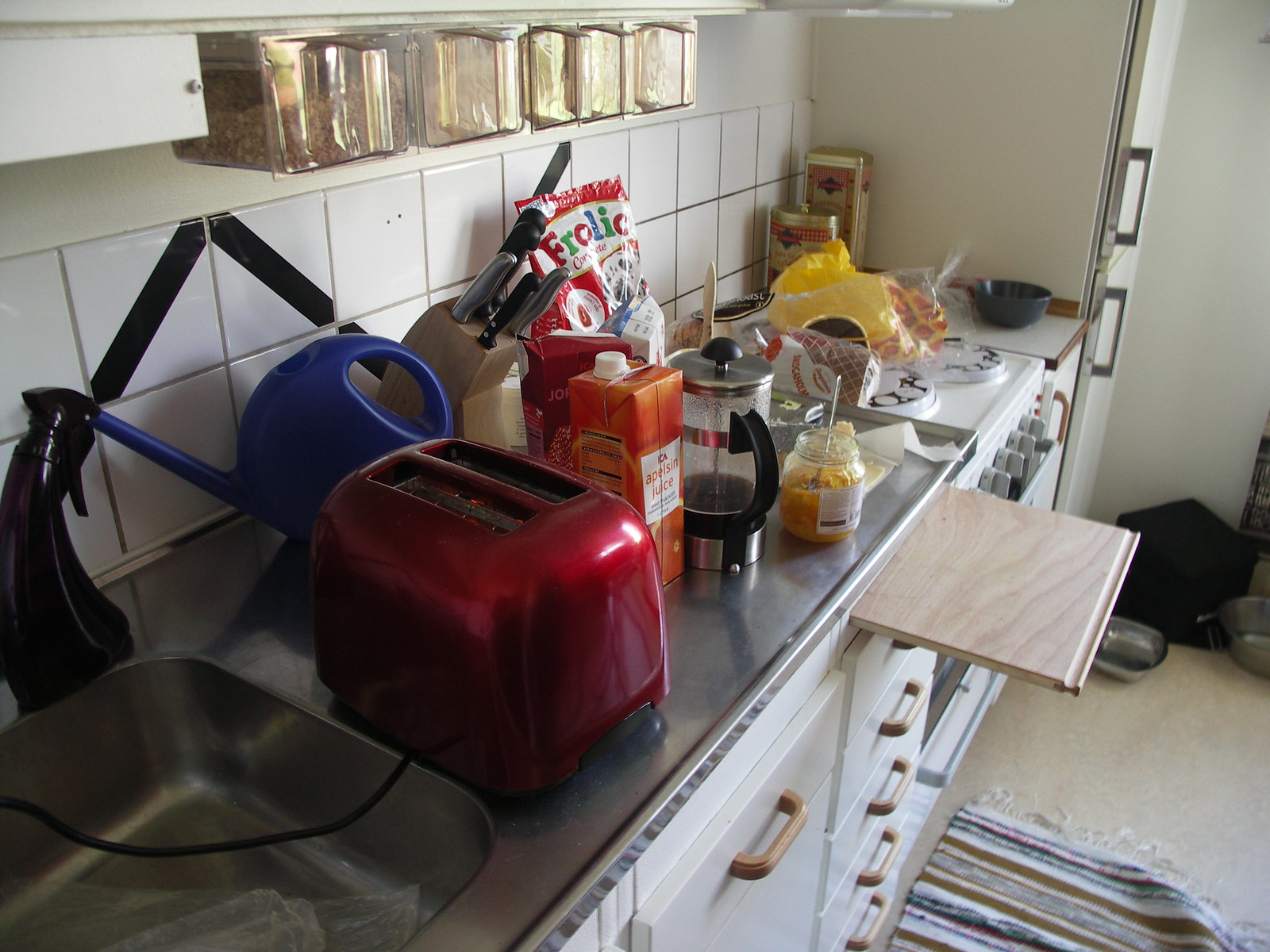In the image, a kitchen table is prominently displayed, cluttered with various items. Starting from right to left: 

- A stainless steel sink is partially visible.
- Next to it is a red toaster, capable of toasting two slices of bread.
- Adjacent to the toaster is a knife block holding several knives.
- A blue plastic container is placed nearby.
- Several bottles, likely for cooking oils or sauces, are scattered across the table.
- A coffee strainer sits next to an open jar filled with a yellow substance, a fork inserted into it.
- In the background, a plate with a stack of waffles is visible.

On the left side of the image, the floor is white, and a fabric mat with brown and blue stripes slightly creeps into view. The kitchen cabinets have brown handles, and the white walls are adorned with white tiles near the sink area, where several canisters filled with various items are placed.